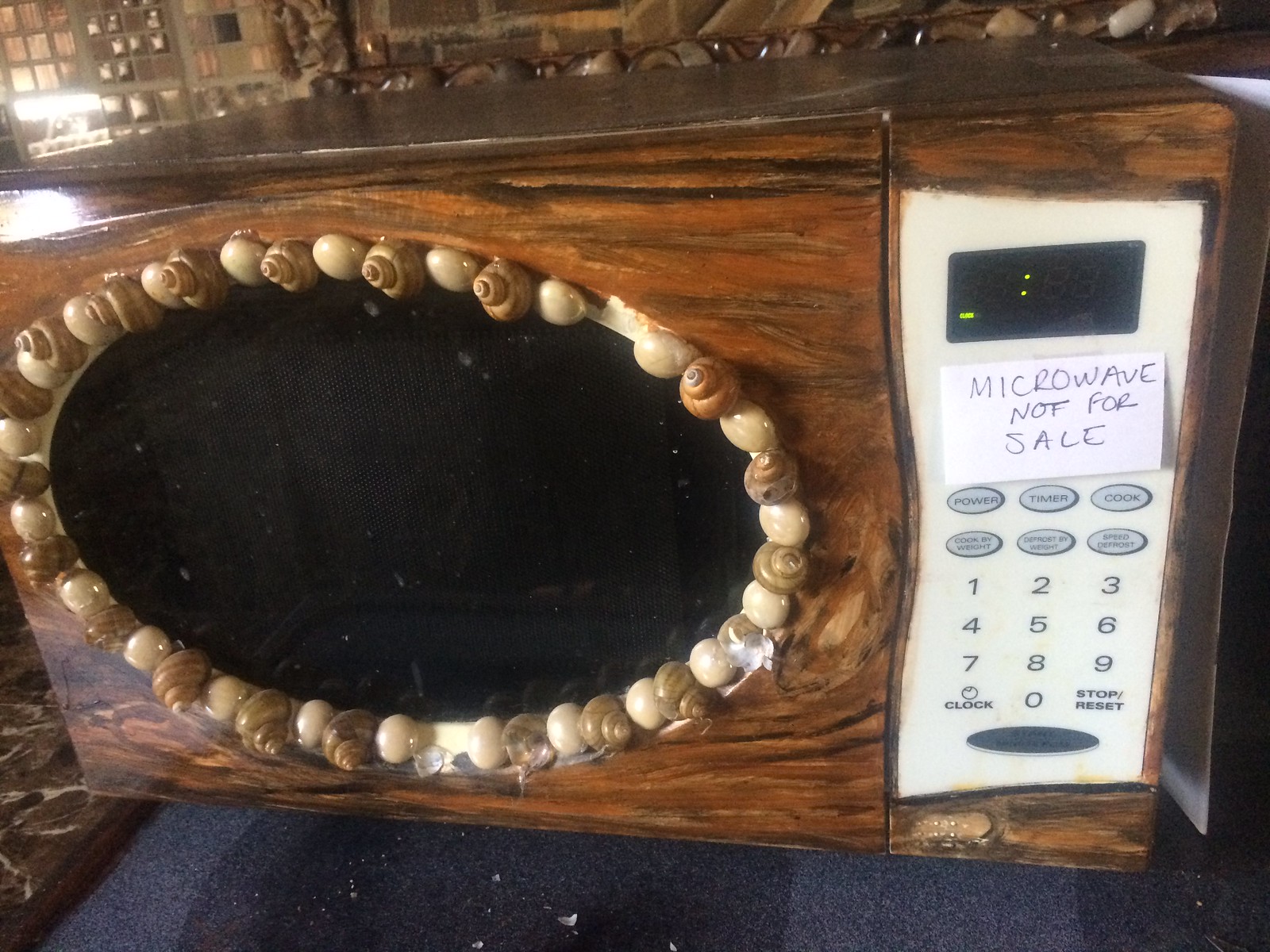This photograph captures a uniquely modified microwave oven set on a table draped with a blue cloth. The microwave, originally a standard model possibly white plastic, has undergone a complete transformation into a striking art piece with a beachy theme. The exterior has been meticulously covered in a rich, weathered walnut brown material with black and cream accents, giving it a distressed, sea-weathered appearance. The most eye-catching feature is the front door, which has been overlaid with a thin sheet of real wood. An oval window at the center of the door is creatively adorned with alternating brown and cream snail shells, and a few pieces of sea glass, most of which form a charming border around the window, though one or two shells are missing. The control panel, partially visible, features a digital display showing just two dots and a small word in the bottom left corner, indicating its digital nature. A handwritten sign on the panel reads, "microwave not for sale." The scene suggests the microwave is in a store or a shop, with a small lamp visible in the background, enhancing the cozy and artisanal atmosphere of the setting.